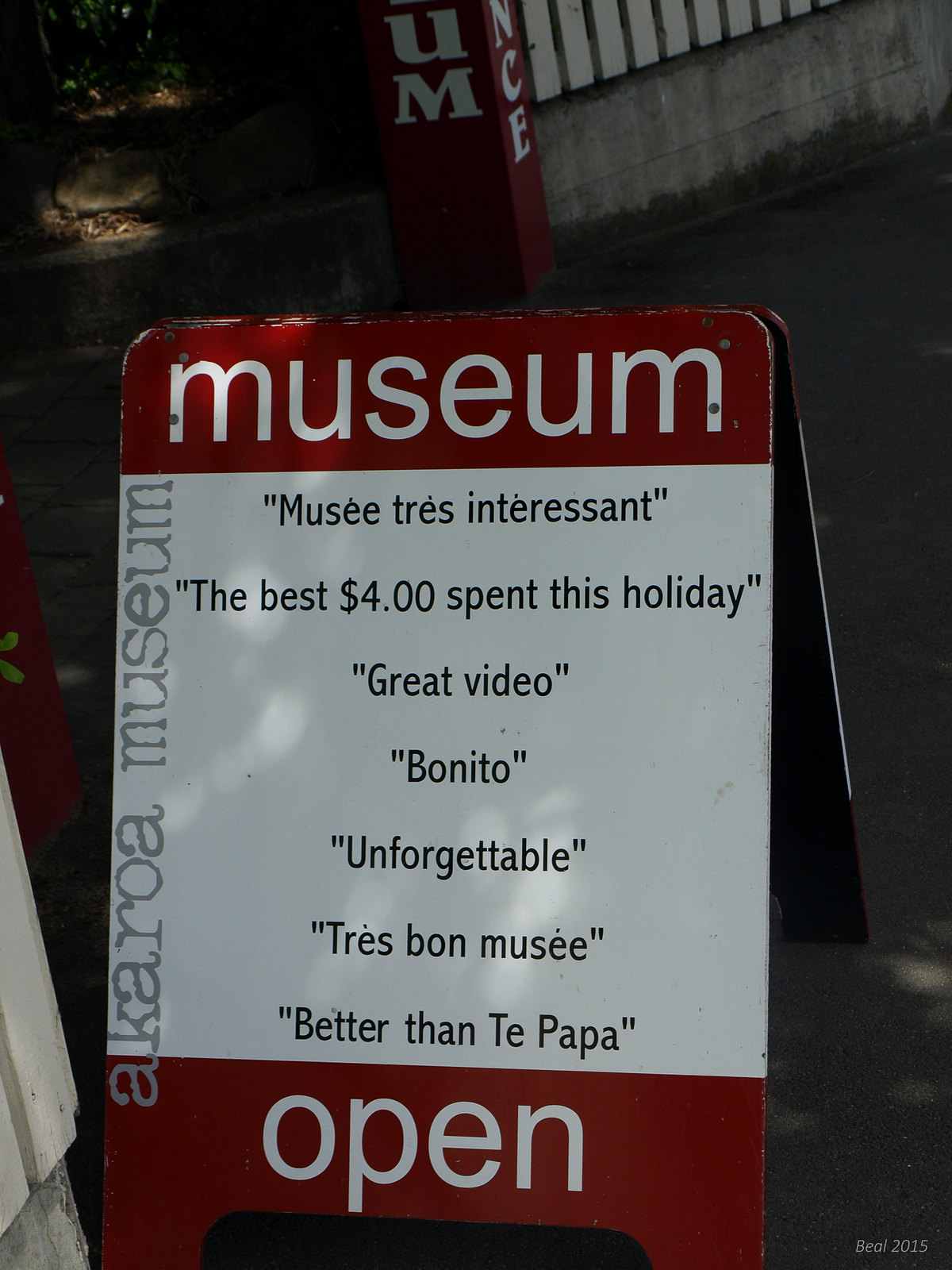This photograph showcases an A-frame sidewalk sign situated outdoors, likely near the entrance of a museum. The sign features prominent red borders at the top and bottom, with the top section displaying the word "Museum" in white text on a red background, and the bottom section stating "Open" in matching style. The central portion of the sign is white with various text elements in black. In black text, one line reads, "The best four dollars spent this holiday," followed by "Great video, bonito, unforgettable." On the left side of the white background, there is vertical gray text running from bottom to top that reads "Akaroa Museum." Some portions of the text in the middle appear to be in a foreign language, contributing to the overall informative and inviting appearance of the sign.